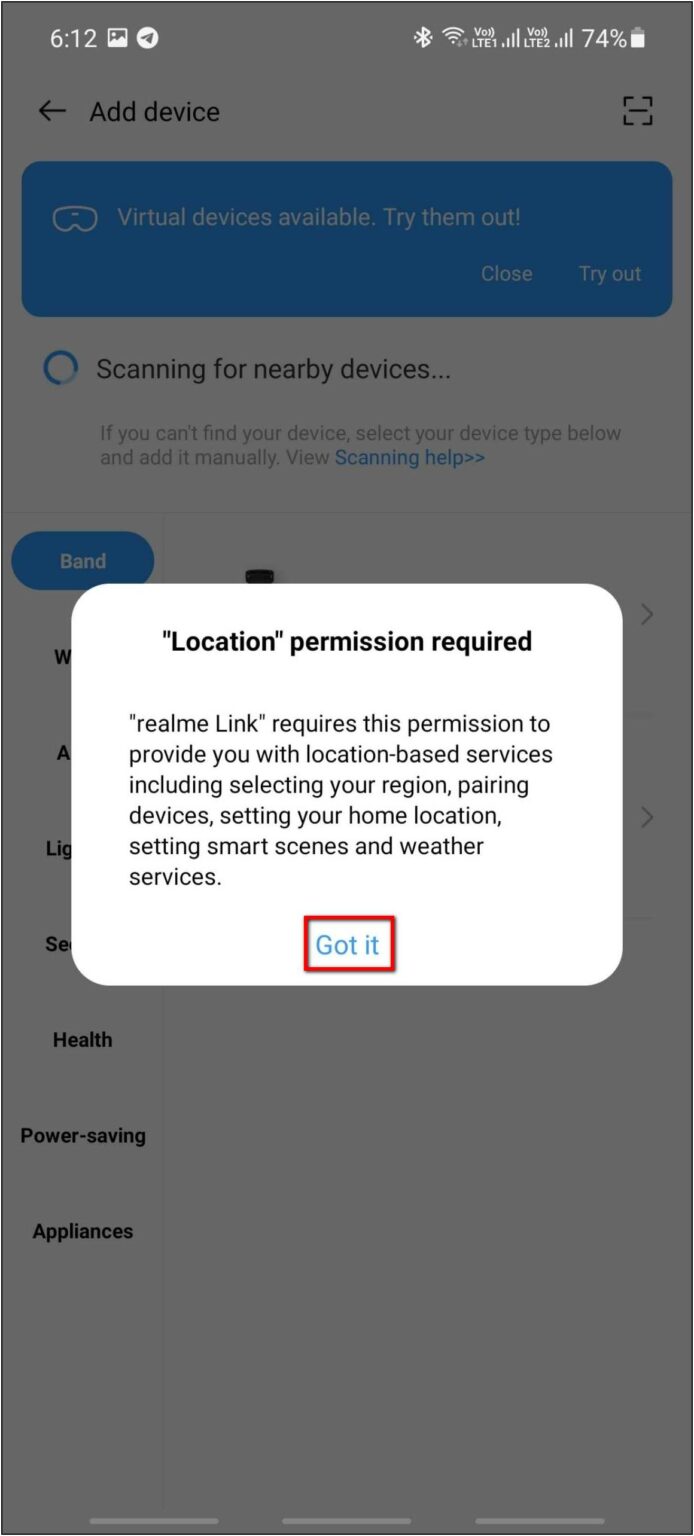The image depicts a user interface screen for adding a new device within the Realme Link app. Front and center, a white pop-up box with rounded edges is displayed, requiring the user to grant location permission. The dialog within the pop-up reads: "Location Permission Required." Below this header, it states, "Realme Link requires permission to provide you with location-based services, including selecting your region, pairing devices, setting your home location, and configuring smart scenes and weather services."

The pop-up dialog offers an acknowledgment button labeled "Got it" within a red-bordered box positioned centrally at the bottom. The background behind the pop-up is grayed out, indicating it is inactive until the required action is completed.

At the top of the underlying screen, the heading "Add Device" is prominently displayed. Below this, a blue button labeled "Virtual Devices - Try them out" is available for users to explore simulated devices. In the bottom-right corner of this section, there’s an option labeled "Close and Try It," alongside a spinning blue buffering icon indicating that the app is actively scanning for nearby devices. If no device is found, an instruction reads: "If you can't find your device, select your device type below and add it manually."

Further down, a message offers users help with their setup, followed by a row of blue buttons for making various selections. These buttons are partially obscured by the pop-up but visibly include categories such as "Health," "Power Saving," "Appliances," and other options, totaling seven different selections.

The interface sits against a clean, white background, complemented by a blue box for virtual devices, reinforcing a simple and modern design language. At the very top of the screen, the status bar indicates it is 6:12, with 74% battery life remaining, two LTE signals, and an active Bluetooth connection.